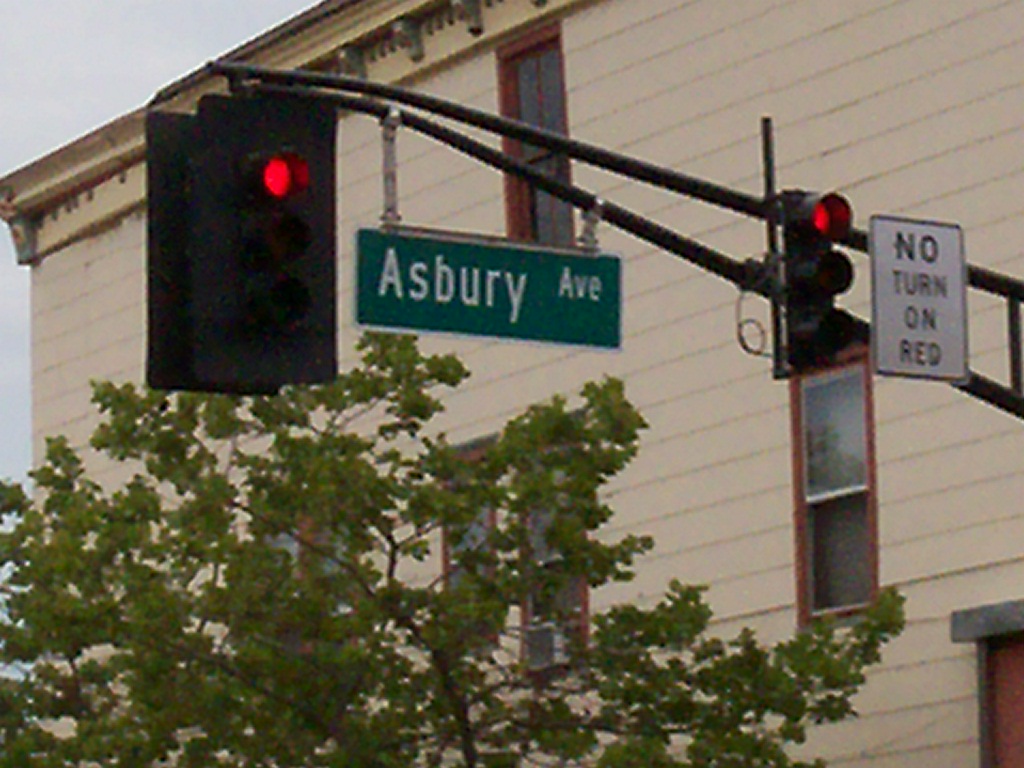This real-life photo captures a close-up view of a traffic light at the intersection of Asbury Avenue. The image focuses on the traffic lights, resulting in a somewhat pixelated and blurry effect. Two traffic lights are mounted on poles extending from the corner, both displaying red signals. Attached to the setup is a dark green sign with white text reading "Asbury Avenue," alongside a rectangular "No Turn on Red" sign, featuring black letters on a white background and framed in black. 

In the background, a large, three-story building is visible, viewed from a low angle that highlights the upper left corner of the structure. The scene also includes the top portion of a green-leaved tree, suggesting lush foliage. The top left corner of the image reveals an overcast sky, subtly indicating daytime conditions. Overall, the image blends urban infrastructure with elements of natural and architectural interest.